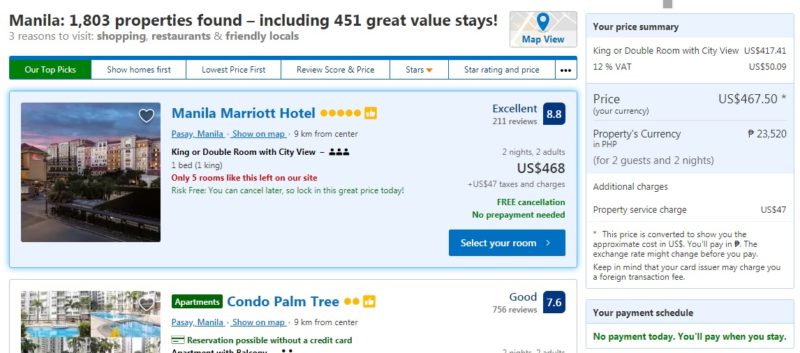This screenshot from a travel booking website features a list of 1,803 properties in Manila, including 451 highly rated value stays. At the top, there's a "Map View" button and a section highlighting three reasons to visit Manila: shopping, restaurants, and friendly locals.

A navigation bar with various sorting options is displayed, including "Our Top Picks" (highlighted), along with "Show Homes First," "Lowest Priced First," "Review Score and Price," and "Stars, Star Rating and Price."

The primary listing showcased is for the "Manila Marriott Hotel." The featured room option is a King or Double Room with a city view. Availability is limited with only five rooms left. The booking is risk-free with free cancellation and no prepayment required. The hotel has excellent reviews, averaging a score of 8.8 from 211 reviews. The price for a two-night stay for two adults is $468, plus $47 in taxes and charges, totaling $515. The payment can be made on arrival.

On the right-hand side, a price summary breaks down the costs: the room is priced at $417.41, with an additional 12% VAT ($50.09), bringing the total to $467.50 USD, equivalent to PHP 23,520. The property service charge of $47 is also highlighted. The payment schedule indicates that no payment is required at the time of booking and will be collected upon check-in.

Partially visible beneath this listing is another for "Condo Palm Tree," but details are cut off.